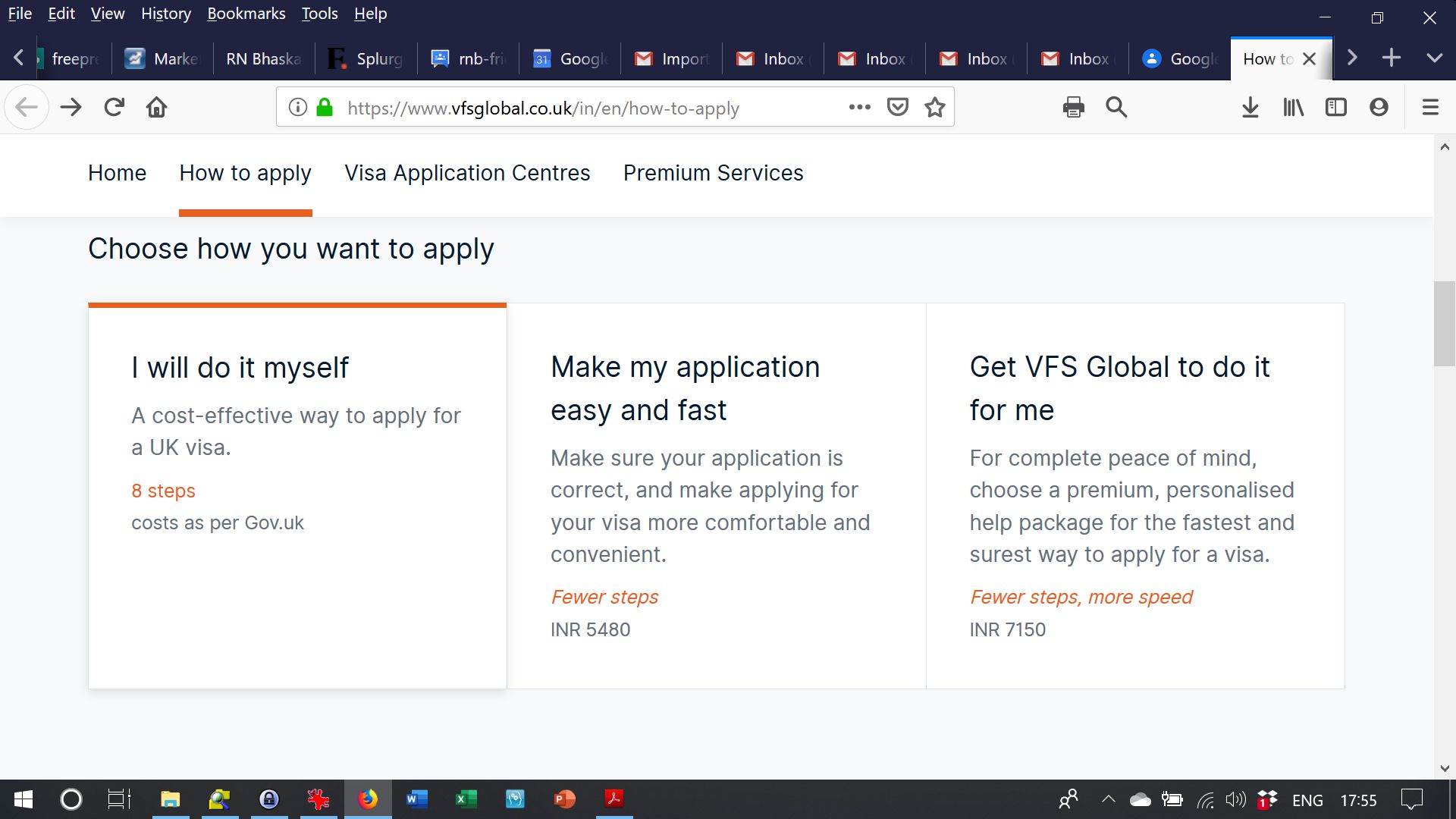In the image, a Mozilla Firefox browser window is open on a computer. The Mozilla Firefox icon is highlighted on the taskbar at the bottom, alongside other application icons such as Adobe Reader, Microsoft Excel, File Manager, and a VPN service.

The browser's main page is white and displays the webpage "vfsglobal.co.uk" under the section "How to Apply." At the top part of the webpage, there are four navigation tabs: "Home," "How to Apply" (which is currently selected and highlighted with an orange underline), "Application Centers," and "Premium Services."

Below the main navigation, the page presents three application method options, each described in separate sections:
1. **"I will do it myself"**: A cost-effective way to apply for a UK visa, following an 8-step course as per gov.uk guidelines.
2. **"Make my application easy and fast"**: Ensures the application is correct and simplifies the visa applying process, reducing the number of steps to 5 and costing £54.80.
3. **"Get VFS Global to do it for me"**: Offers a premium, personalized help package for the fastest and most efficient application process, reducing the steps to just 2, at a cost of £71.50.

The text on the webpage is black, creating a clear contrast against the white background, making the information easy to read.